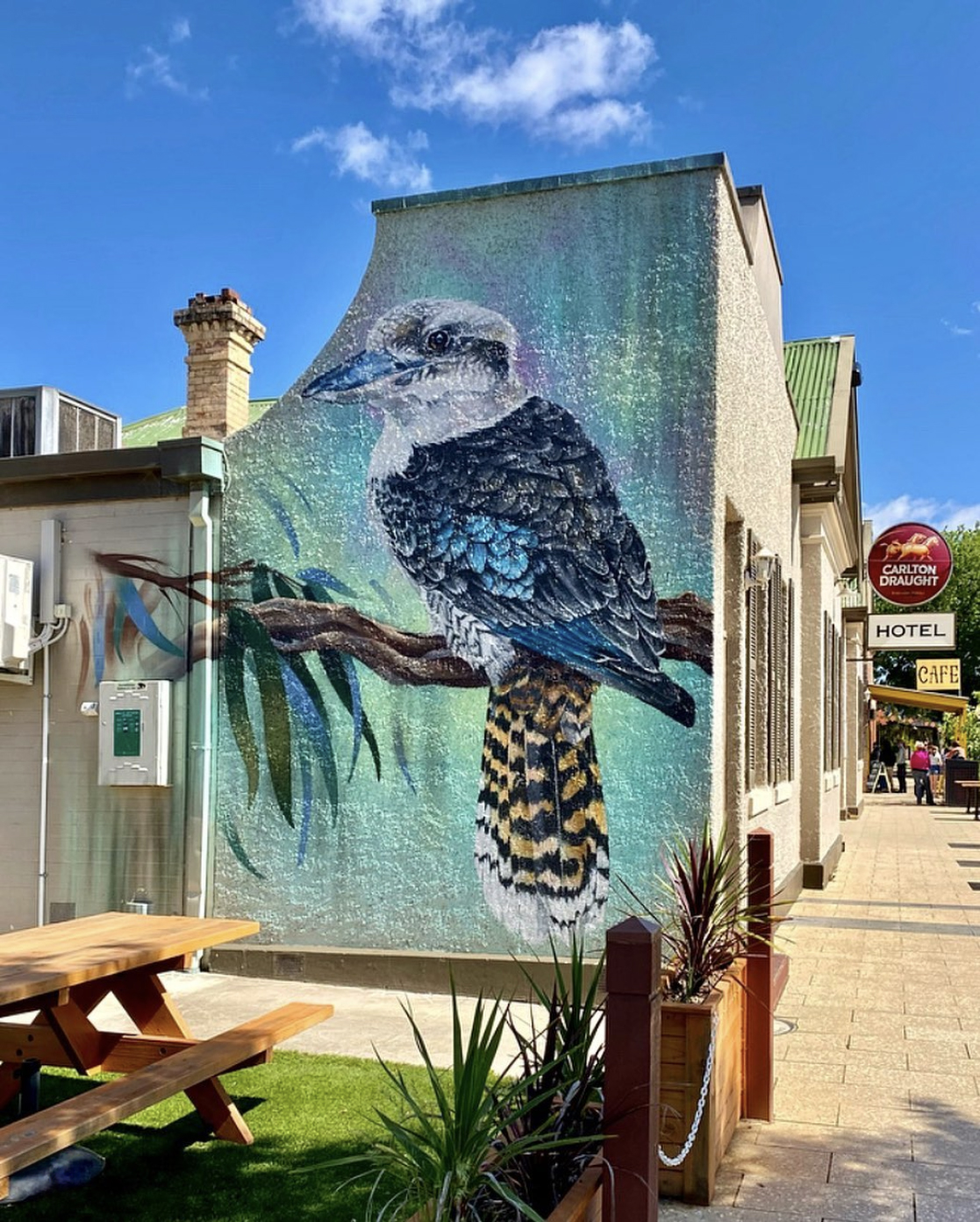This color photograph captures the vibrant side of a gritty urban building, likely a pub, situated next to the Carlton Drott Hotel and a nearby cafe. The main feature is an expansive mural covering the entire wall. The artwork portrays a detailed depiction of a kookaburra perched on a gum tree branch with small, wilted eucalyptus leaves hanging from the left side. The bird, predominantly painted in various shades of blue, has dark blue feathers with lighter blue near the tips of its wings, a striking white head and neck, a distinctive black stripe near its eye, and a long blue and white beak. Notably, its tail feathers are adorned with tiger-like stripes. The mural's palette includes striking blues, yellows, and purples, enhancing its visual appeal. Below the mural, there is a fenced-off picnic table area with long benches, providing a space for patrons to sit and enjoy their drinks, likely beer from Carlton Draft, in an outdoor setting.